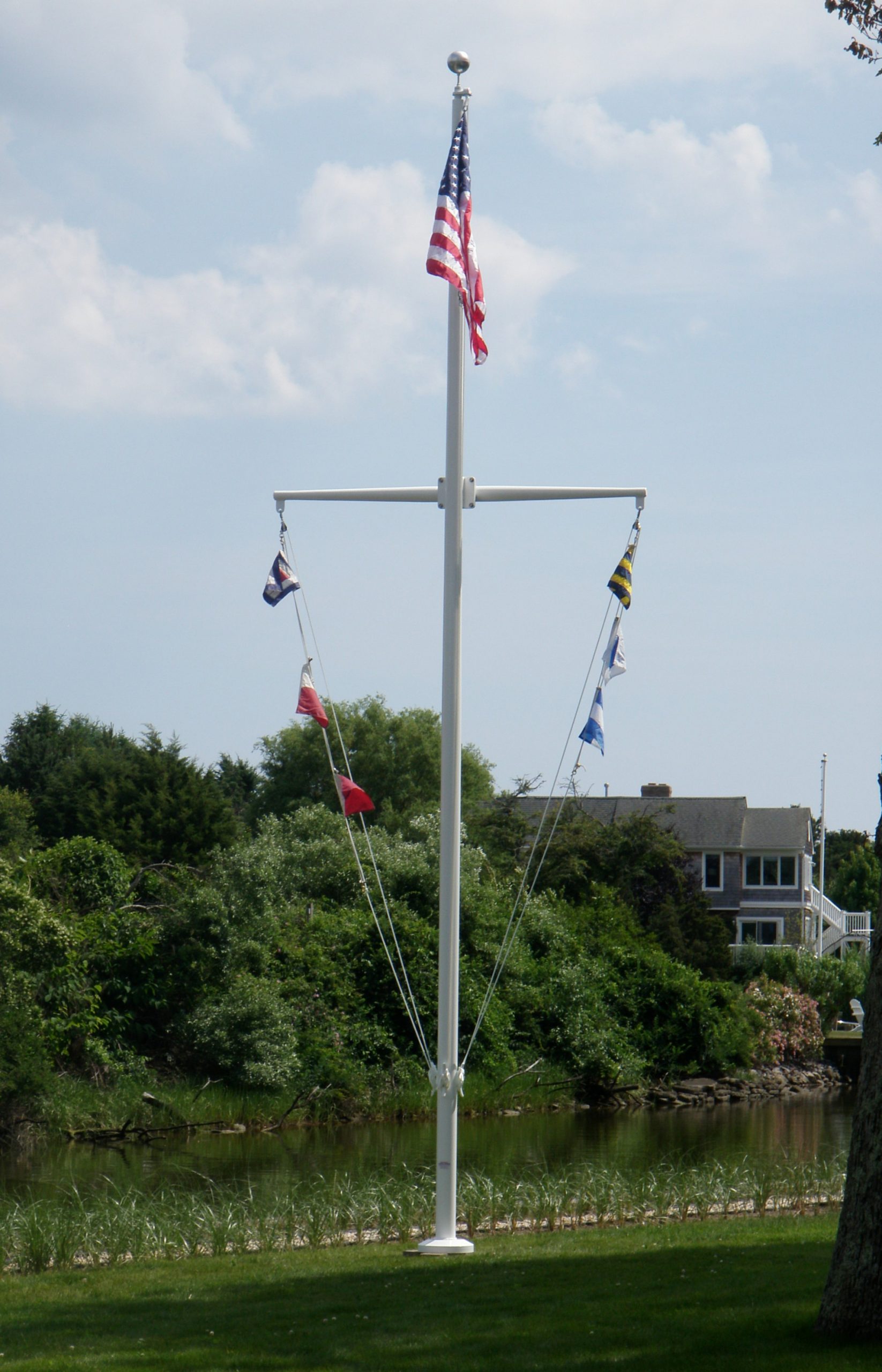In this picturesque image, the focal point is a tall, white maritime flagpole topped with a silver ball and an American flag. Below the American flag, the pole branches out into a T-shape, supporting six smaller flags arranged in an upside-down triangle, each in different colors, including red, blue, and yellow. The flagpole is positioned in a lush, green landscape with a shady foreground of grass and a murky body of water—possibly a river—lying just behind. Beyond the water, there are dense trees and a house, which appears to be a visitor center or a residence, displaying a gray or blue hue. The backdrop features a clear, blue sky dotted with a few wispy clouds, suggesting a calm, windless day. The strings on the flagpole, used to raise and lower the flags, can be seen tied off near the base of the pole. The scene captures a serene and scenic setting with the well-maintained greenery, still water, and the striking arrangement of flags.